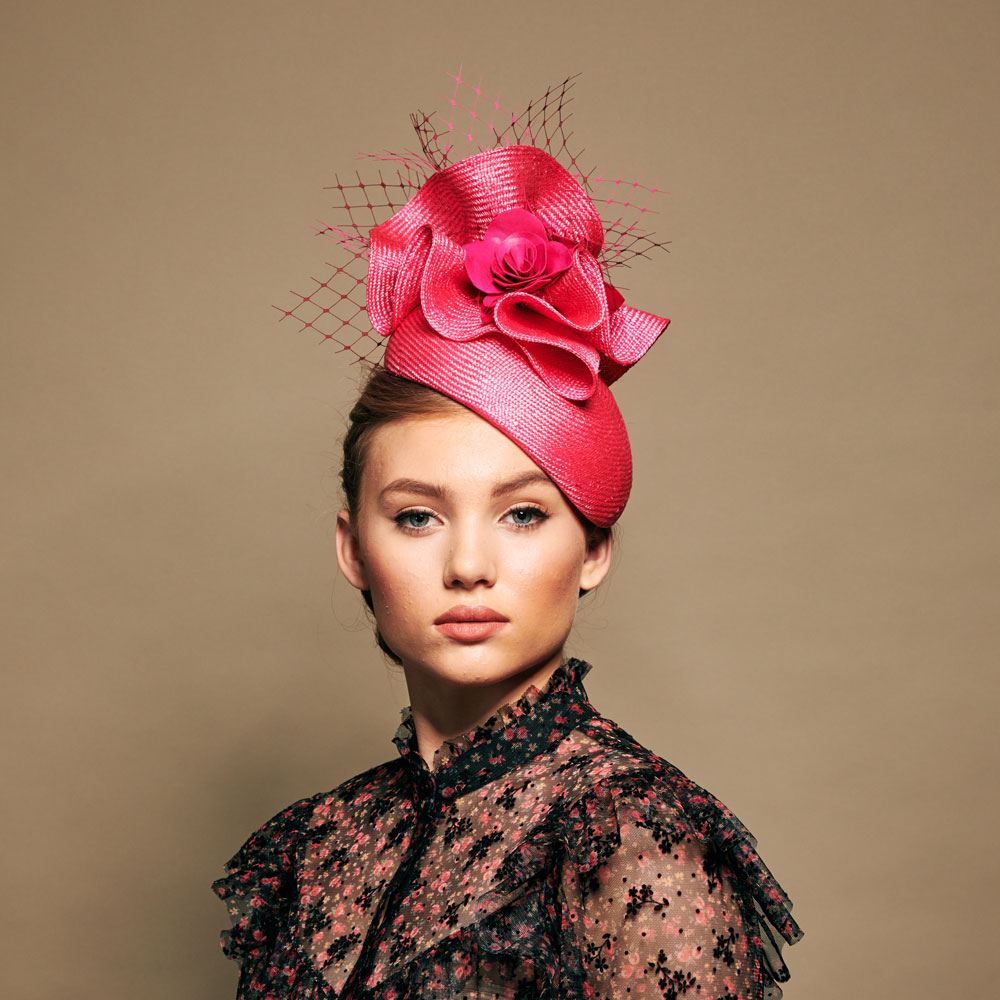This fashion portrait features a lone Caucasian model standing against a plain tan background, allowing her attire and presence to dominate the scene. The model, with her auburn hair neatly pulled back and up, sports a striking red satin dress hat. The hat boasts intricate folds and loops of fabric, creating the appearance of delicate flower petals across the top of her head. Interwoven within these folds, red netting adds an additional layer of texture and sophistication. The model's smooth, youthful face is accentuated with subtle makeup, complementing her blue eyes.

Her dress is a stunning black lace creation that exudes an antique charm. The high-collared dress, fastened at the front with either a button or a zipper, features intricate lacework with embroidered black flowers and polka dots layered over a pink floral print. A tank top or slip is visible underneath, enhancing the modest yet elegant appeal of the semi-transparent lace. The gauzy shoulders and arms of the dress contribute to its delicate aesthetic, while the frilly lace collar and accents on the shoulders complete the old-fashioned yet timeless look.